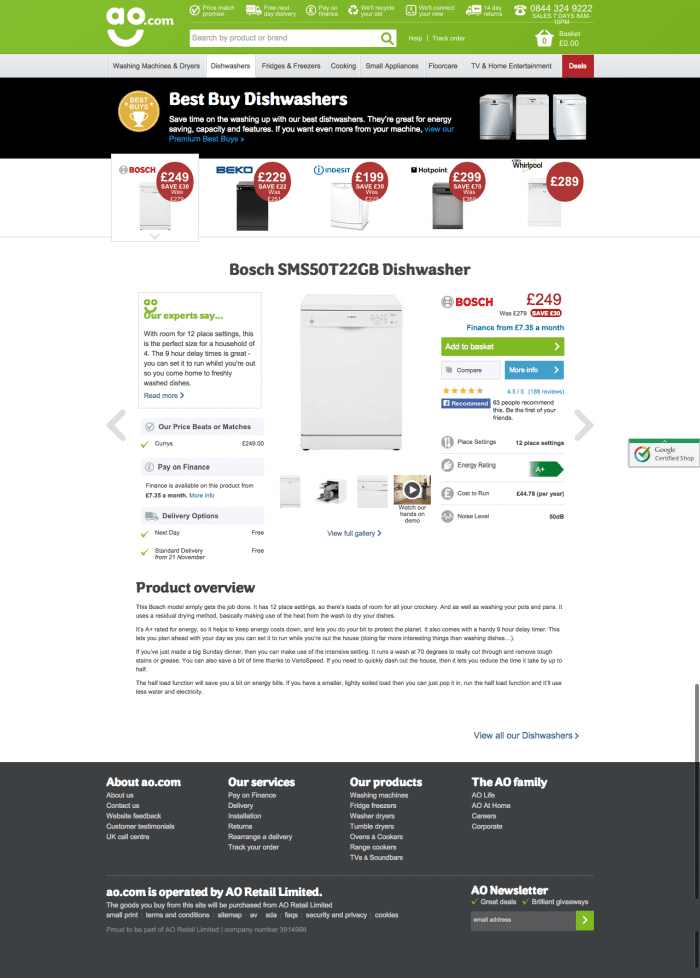The image displays the homepage of AO.com, an online appliance retailer. At the top, there's a prominent search field labeled "Search by product or brand." Additional features highlighted include "Price Match," "Pre-Next Day Delivery," "Prioritized," and options to "Recycle Your Old," "Pay on Finance," or "Connect Your New" appliance. The site offers a "14-Day Returns" policy and provides a contact number, 0844-324-9222, for sales inquiries available seven days a week from 5 AM to 10 PM. The shopping basket currently shows a balance of £0.00. A highlighted section promotes "Best Buy Dishwashers," emphasizing their ability to save time on washing up, energy efficiency, capacity, and features. The message concludes with a call to explore even higher-performance options, referred to as "Platinum Best Buy."